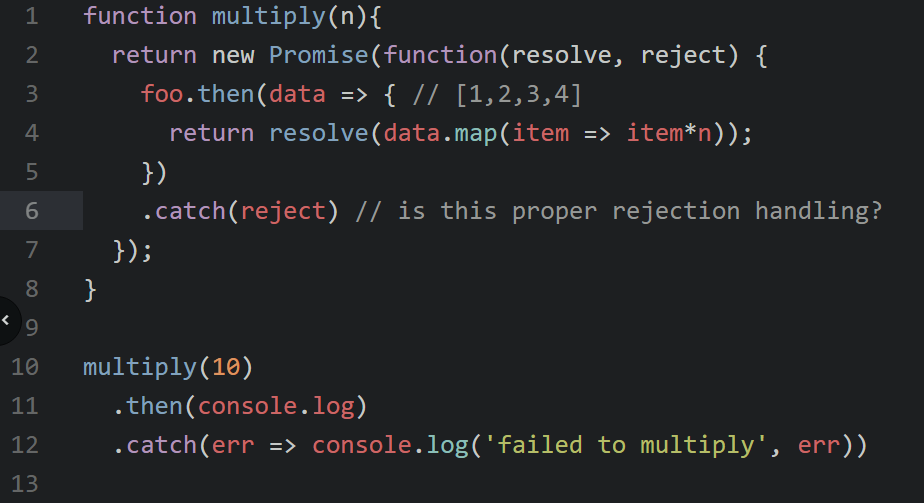The image depicts a segment of code on a dark-themed code editor interface. The lines of code are numbered vertically from 1 to 13 along the left side of the screen. The syntax highlighting uses different colors to differentiate various elements of the code. 

- Line 1 features the declaration of a function named `multiply`, where the keyword `function` is highlighted in purple and `multiply` in blue.
- Lines 2 through 8 contain additional code that cannot be discerned from the verbal description provided.
- Lines 9 and 13 are completely empty.
- On line 10, the word `multiply` appears again in blue, followed by `(10)` in orange, with the number `10` being the only orange element in the entire image.
- On line 12, a string enclosed in parentheses reads "part of the sentence has failed to multiply," highlighted in yellow. This yellow text is unique to this line.

The entire code segment sits on a black background, typical of dark-mode themes in coding environments.